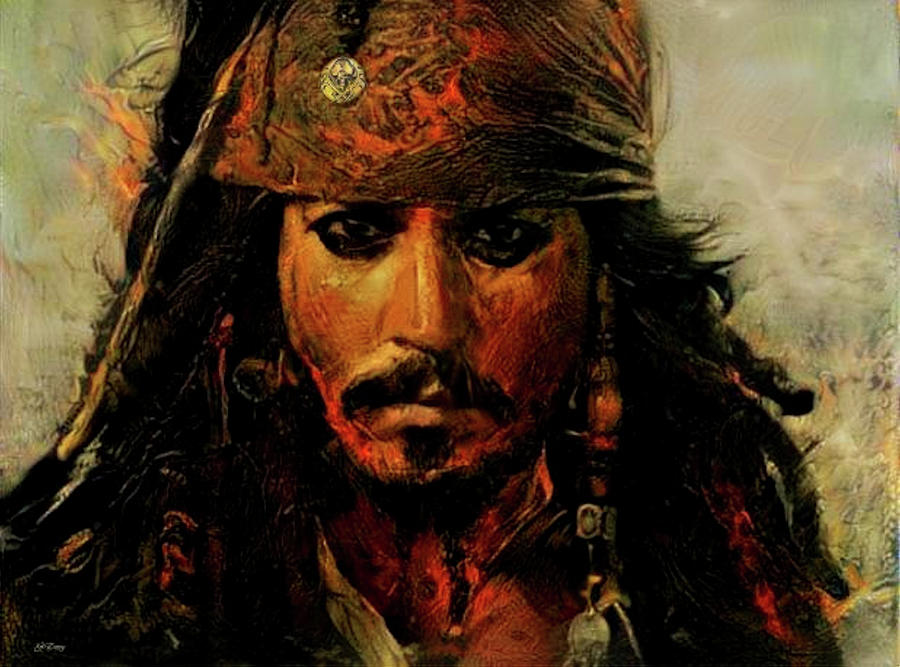This is a detailed painting of Captain Jack Sparrow from the Pirates of the Caribbean, clearly recognizable as Johnny Depp's iconic character. The portrait focuses on his head and a slight bit of his chest. He is staring directly ahead, wearing a distinctive red bandana with a gold pendant attached. His long, dreadlocked black hair is tied up in the back, adorned with beads and silvery metal pieces, including beaded tassels and jewelry. Sparrow's characteristic facial features are meticulously portrayed: prominent black eyeliner or mascara encircles his eyes, and he sports a mustache paired with a beard styled in a small soul patch and two knots. His face has warm tones of red and orange, giving a tanned appearance. The background of the painting is somewhat blurry on the left side, bringing all attention to Jack Sparrow's detailed and expressive visage.